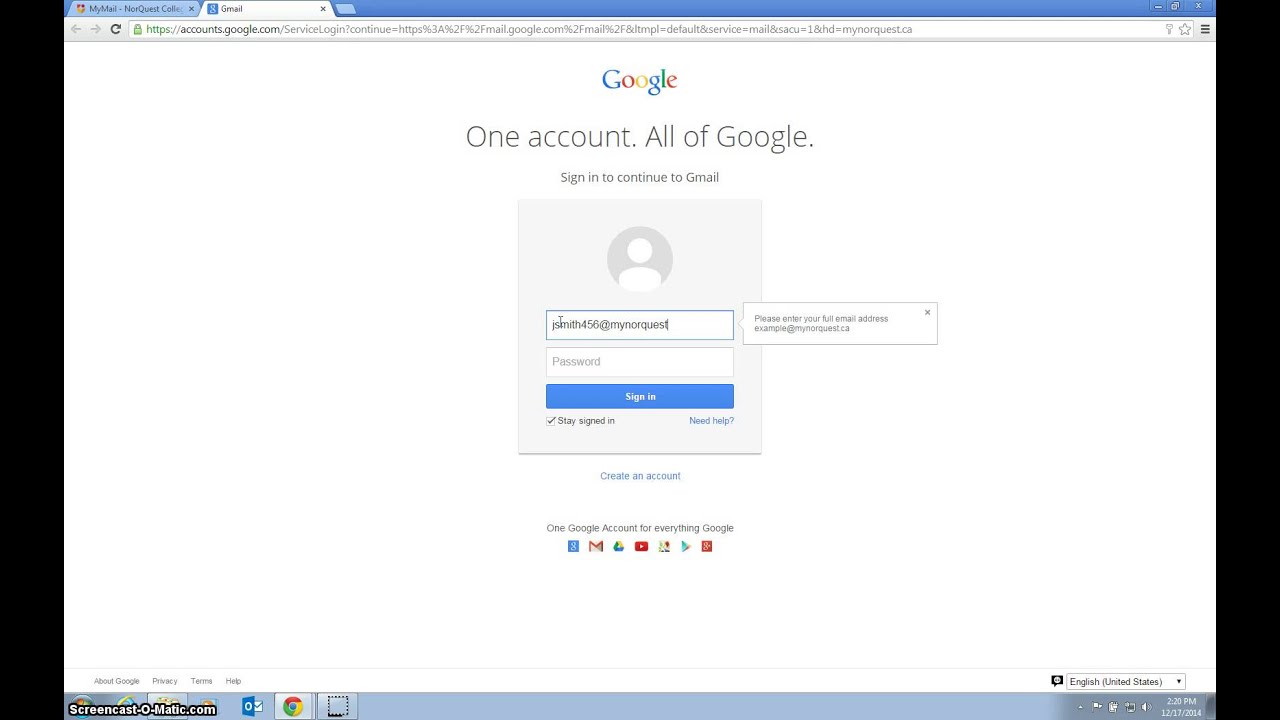The image displays a Google sign-in page. At the top, there is a slightly blurred search bar where something has been entered but is unreadable. The browser interface shows active tab highlights in blue and white. Centrally, the prominent Google logo is presented in its characteristic blue, red, gold, and green colors. Below the logo, the text "One account. All of Google." is rendered in gray.

Directly under this text, a prompt reads, "Sign in to continue to Gmail." Below the prompt, there is a gray box featuring a generic user icon. Adjacent to this icon is a white box containing typed information, likely a placeholder for the username. To the right, another white input field requests the user's credentials.

Under the username field, there is an input field for the password. A blue "Sign In" button is placed underneath, intended for users to click after entering their information.

At the bottom of the page, there is a section referring to "Account" with various colored icons—blue, white, and red—representing different Google services. The footer is light blue, including an image of the Chrome icon and some text in black located at the lower left-hand corner. This intricate layout reflects the standard interface for a Google account sign-in page.